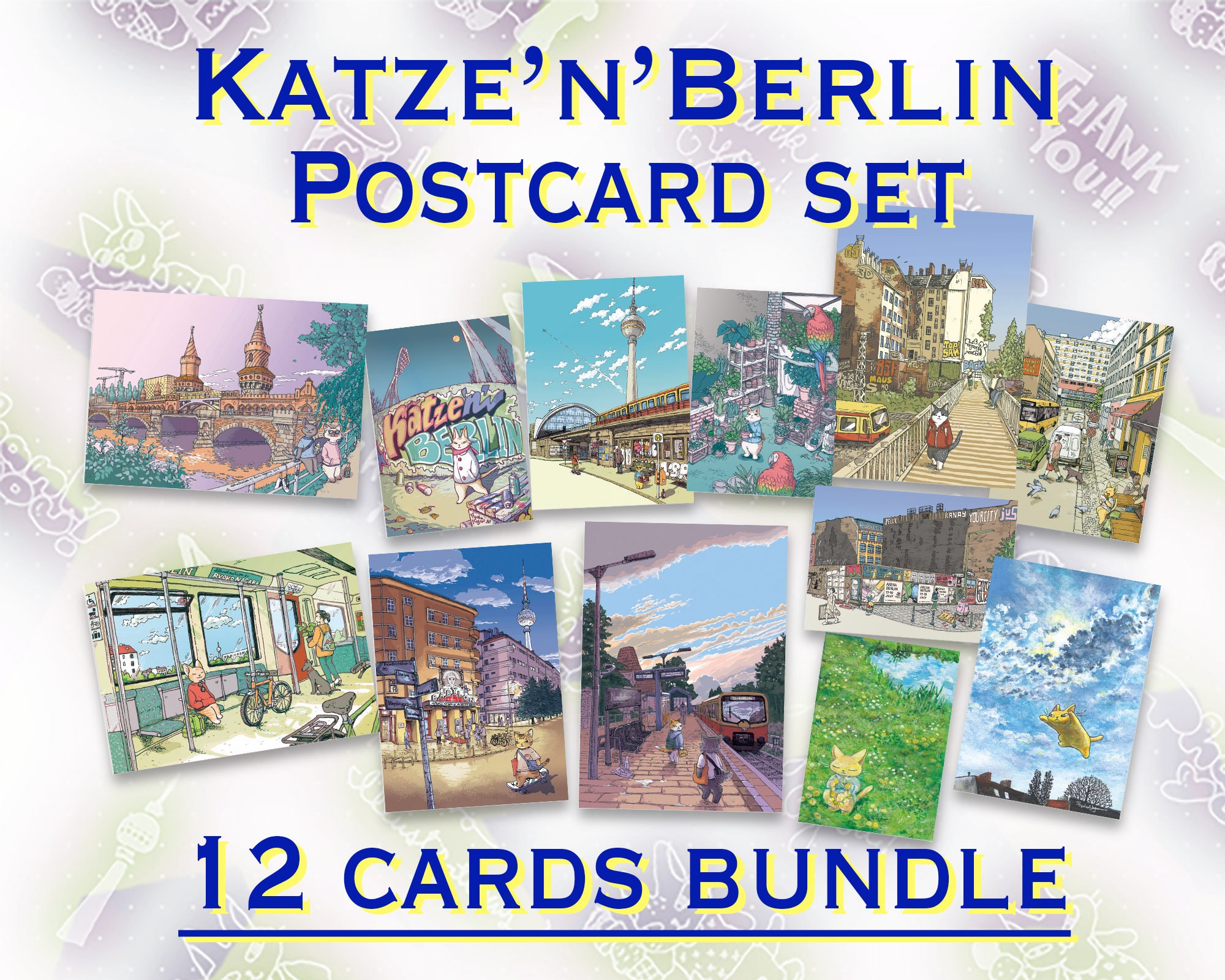The image is an illustrated advertisement for the "Katzen in Berlin" postcard set. At the top, dark blue lettering on a white background reads "Katzen in Berlin," flanked by the word "thank you." Below, twelve colorful, comic-style postcards, arranged in two rows, depict the main character, Katzen, a cat, in various iconic locations around Berlin. Notable scenes include Katzen on a bridge over a river with twin towers, inside a subway car with a bicycle, riding a scooter down a street, waiting at a railway station, relaxing in a grassy field, and flying through a blue sky. Additional settings show Katzen in a bustling urban area, walking on a wooden boardwalk, shopping, visiting a water park, sitting on a park bench, and inside a pet store with birds. The bottom of the image highlights "12 Cards Bundle" in blue letters.